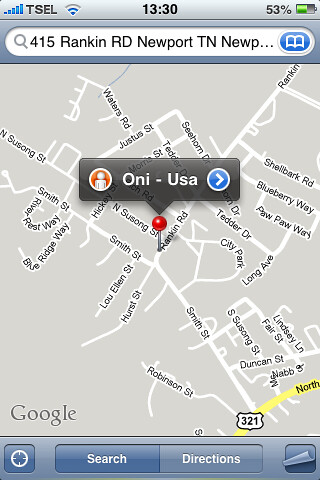The image is a screenshot taken from someone's cell phone, displaying a Google map. At the top of the screen, the status bar indicates the phone is connected to T-Cell with full service and active Wi-Fi connectivity. The time displayed is 13:30, and the battery is at 53%. The map shows a search for the address "415 Rankin Road, Newport, Tennessee," marked with a prominent red pin. The map is detailed, featuring numerous roads, including Pawpaw Way, City Park, and Long Avenue, along with a highway labeled "321" near the bottom right. Additional labels include Oni-USA to the left and Kaling Square to the right. The lower section of the screenshot provides buttons for "Search" and "Directions," with the word "Google" visible in the bottom left corner.